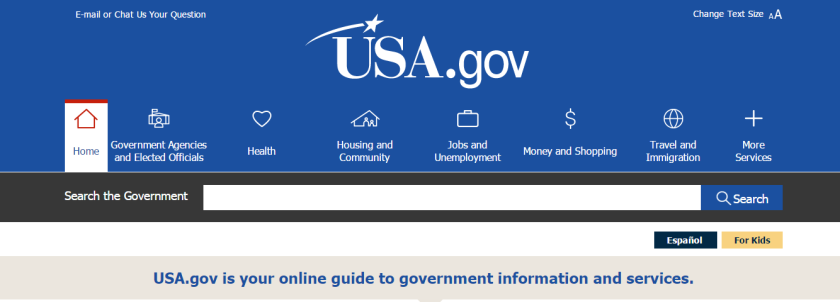The image is a horizontally-oriented rectangular box. The upper portion, which takes up more than half of the entire image, features a blue background with various elements in white text. 

In the top left corner, the text reads "Email or chat," encouraging users to ask their questions. Centered prominently in larger print is "USA.gov" with a decorative shooting star motif over the "U." At the top right, the text says "Change text size."

Below this primary header, there is a row of navigation options highlighted with white backgrounds. These include:
- A highlighted "Home" link.
- "Government Agencies and Elected Officials."
- "Health" accompanied by a heart symbol.
- "Housing and Community" with a house symbol.
- "Jobs and Employment" indicated by a briefcase symbol.
- "Money and Shopping" denoted by a dollar sign symbol.
- "Travel and Immigration" marked with a globe symbol.
- "More Services" signified by a plus sign.

Proceeding down, a black border with white text reads "Search the government." Beneath this, there is a large, empty white search box and a smaller blue box with a white search icon and the word "Search."

Further down, there is a white section including two options: "Espanol," displayed in a black box with white text, and "For Kids," shown in a yellow box with black text.

The final section is a gray box containing the phrase "USA.gov is your online guide to government information and services" written in blue text.